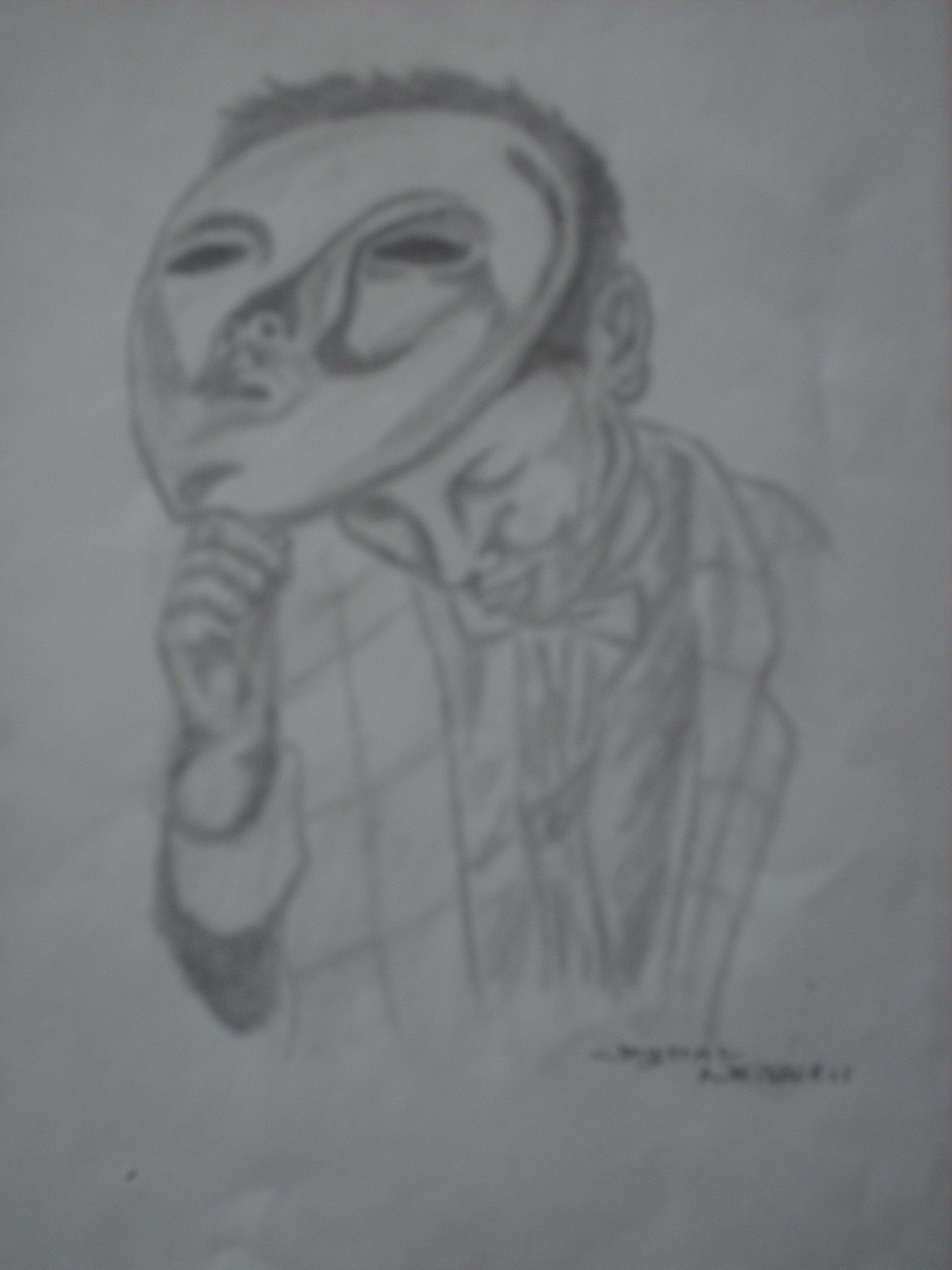A detailed drawing rendered in pencil is set on a gray piece of paper. The artwork portrays a young man with a melancholic expression, his head slightly bent forward. He is captured in the moment of lifting a mask off his face. The mask itself is characterized by distinct features: a round face with long slits for the eyes and an elongated nose. The young man's hand is firmly wrapped around the end of the mask. He is dressed in a long-sleeved white shirt with prominent cuffs and a dark jacket featuring a checkered pattern. Beneath the jacket, a tie is also visible, suggesting a formal attire that contrasts with the sadness conveyed in his demeanor.